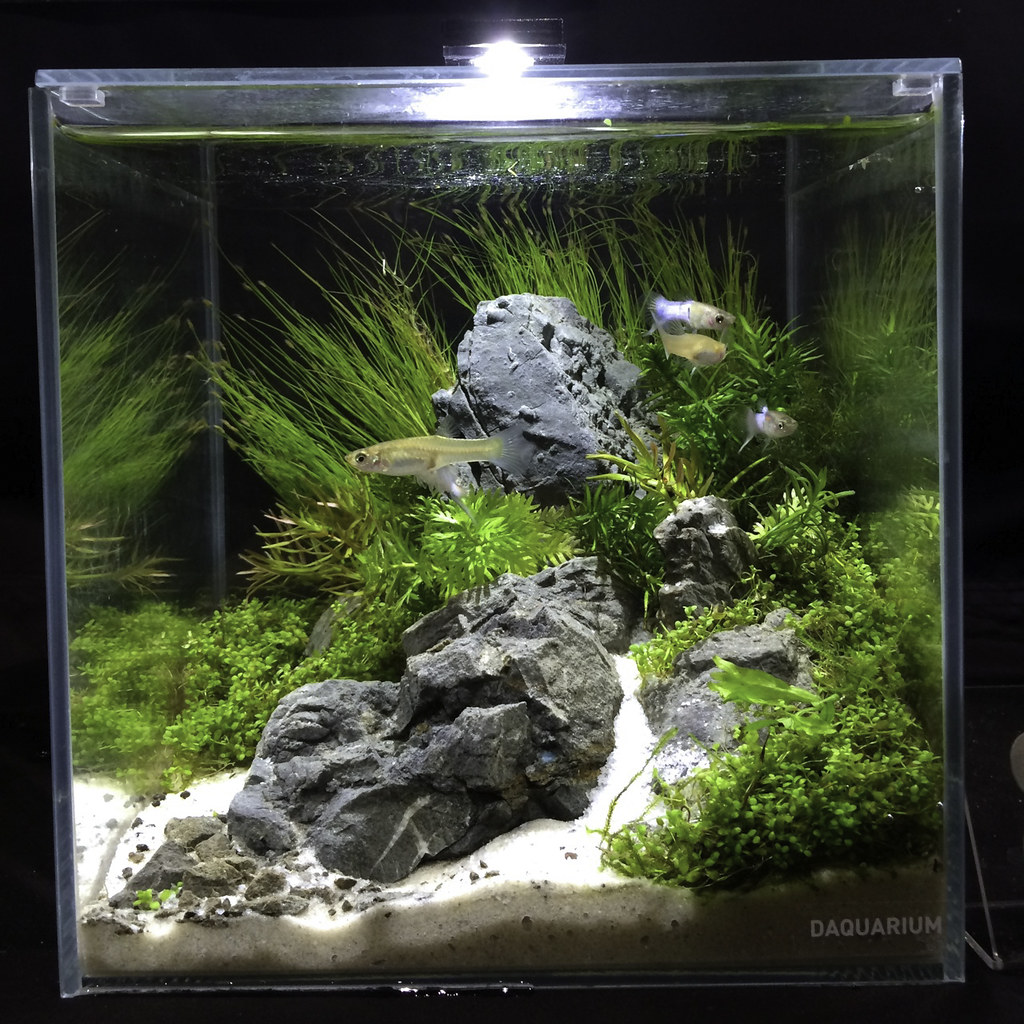This detailed photograph captures a square-shaped aquarium, set against a black background that accentuates the vibrant life within. Illuminating the tank from above is a light that casts a soft glow, highlighting the underwater scenery. Dominating the bottom landscape is a combination of sand and gravel, among which several gray rocks are scattered. In the midst of these rocks, there's an array of aquatic vegetation; some plants bear thin, elongated leaves reaching for the surface, while others are more rounded and provide a lush backdrop.

The foliage is thoughtfully placed around the aquarium, with taller seagrass positioned towards the back and other plants interspersed to offer hiding spots for the inhabitants. Visible among the greenery are four distinct fish: a pale orange fish with a greyish tail swimming to the left, a smaller gold fish, and a grey fish moving in the opposite direction. Additionally, there's another fish, possibly white and partially hidden among the grass, though its features are harder to discern. The aquarium is aesthetically pleasing, inviting the viewer to notice the intricate rock formations and the dynamic aquatic life.

In the bottom right-hand corner, the text "Dad Aquarium" is written in white capital letters, adding a personal touch to this serene underwater tableau.